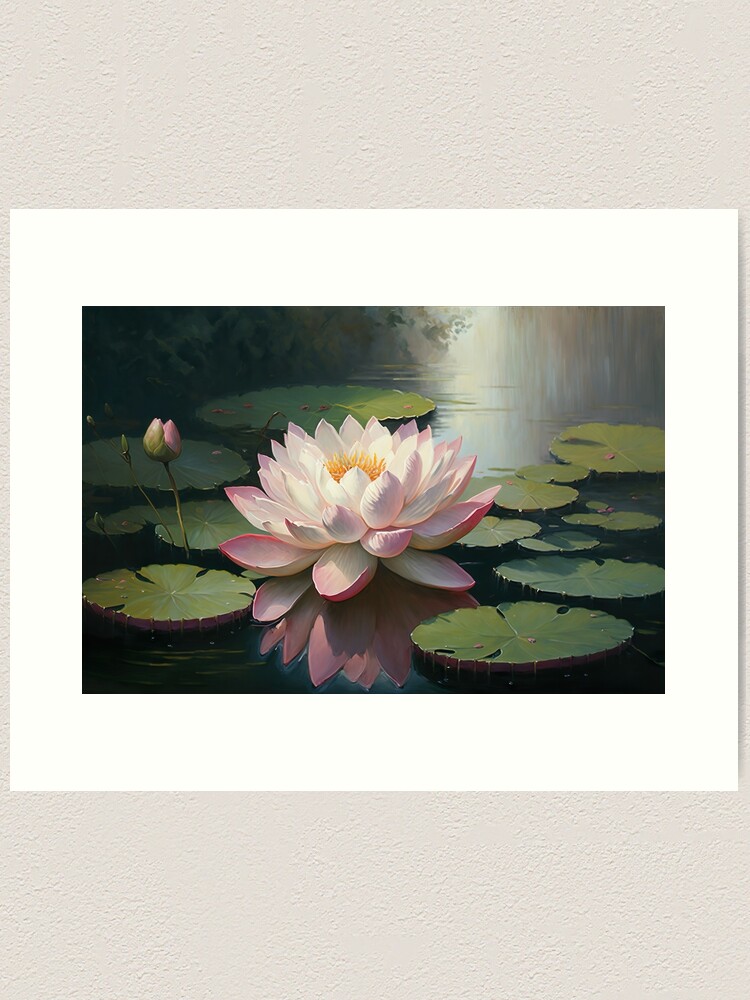A portrait-oriented artwork or photograph is displayed on a textured gray wall, comprising a central image framed by a thick off-white border. The central image portrays a serene aquatic scene with a dark, almost black body of water hosting numerous dark green lily pads. The water is slightly reflective, akin to glass. At the heart of the composition is a striking water lily in full bloom, showcasing a beautiful array of pink and white petals radiating around a vibrant yellow center. To the left of this radiant flower, two buds are visible, one of which is just beginning to open, revealing its pink petals. The light source from the upper right corner casts a soft spotlight, enhancing the flower's delicate beauty and emphasizing its prominence within the picture.